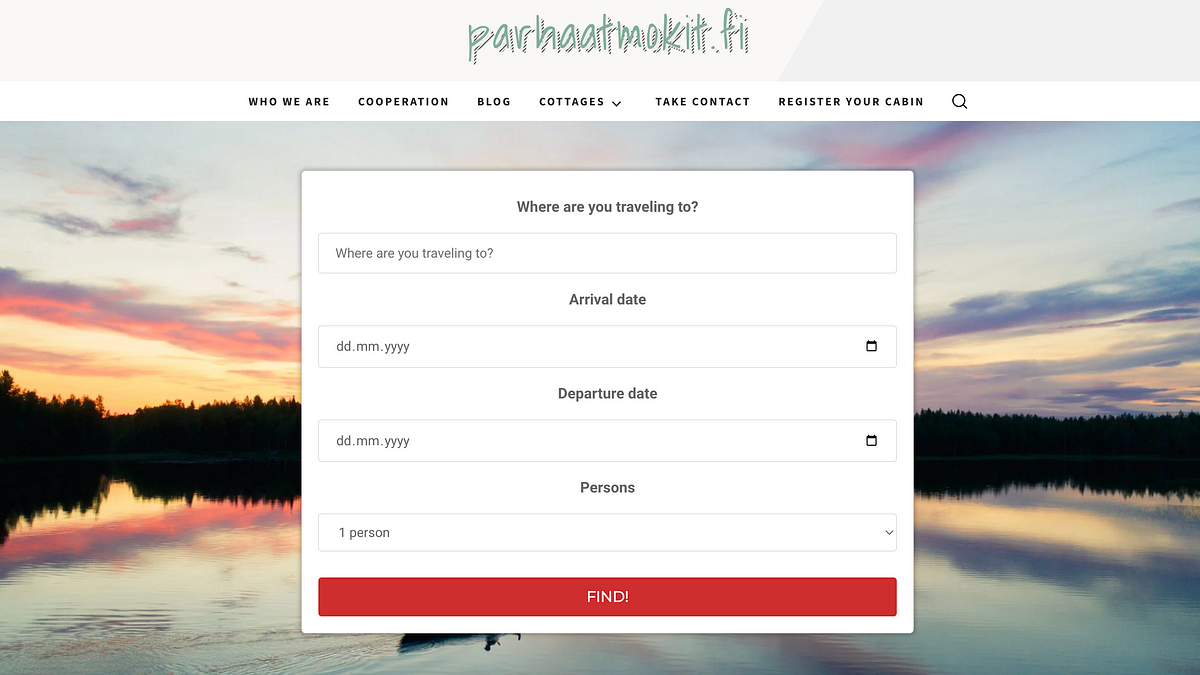This screen capture depicts a website with a clean and organized layout. At the top of the image, there is a header bar in shades of gray and off-white. Prominently displayed within this bar is the website name, "PARHAAT-MOKIT-FI," rendered in a distinctive white, almost olive-hued font.

Beneath the header, there is a series of submenu options in white with black text. These options include tabs labeled "Who We Are," "Corporation," "Blog," and "Cottages," each accompanied by a clickable down arrow. Additional options like "Take Contact" and "Register Your Cabin" are present, along with a black magnifying glass icon for search functionality.

The central section of the screen features a striking background image showcasing a serene body of water. The water's surface reflects an array of pink, purple, and blue hues, creating a mesmerizing gradient from pink and purple on one side to purple and blue on the other. The scene is framed by a dense tree line in the distance and a vibrant sky displaying shades of pink, purple, blue, and a hint of orange.

In the foreground, a white box contains black text that reads, "Where Are You Traveling To?" This box includes input fields for travel details: a field labeled "Where Are You Traveling To?," an "Arrival Date" field formatted as DD-MM-YYYY with a calendar icon, a "Departure Date" field in the same format with another calendar icon, and a "Persons" dropdown menu currently displaying "One Person." At the bottom of the box, a prominent red button with white text invites users to "Find" their desired travel details.